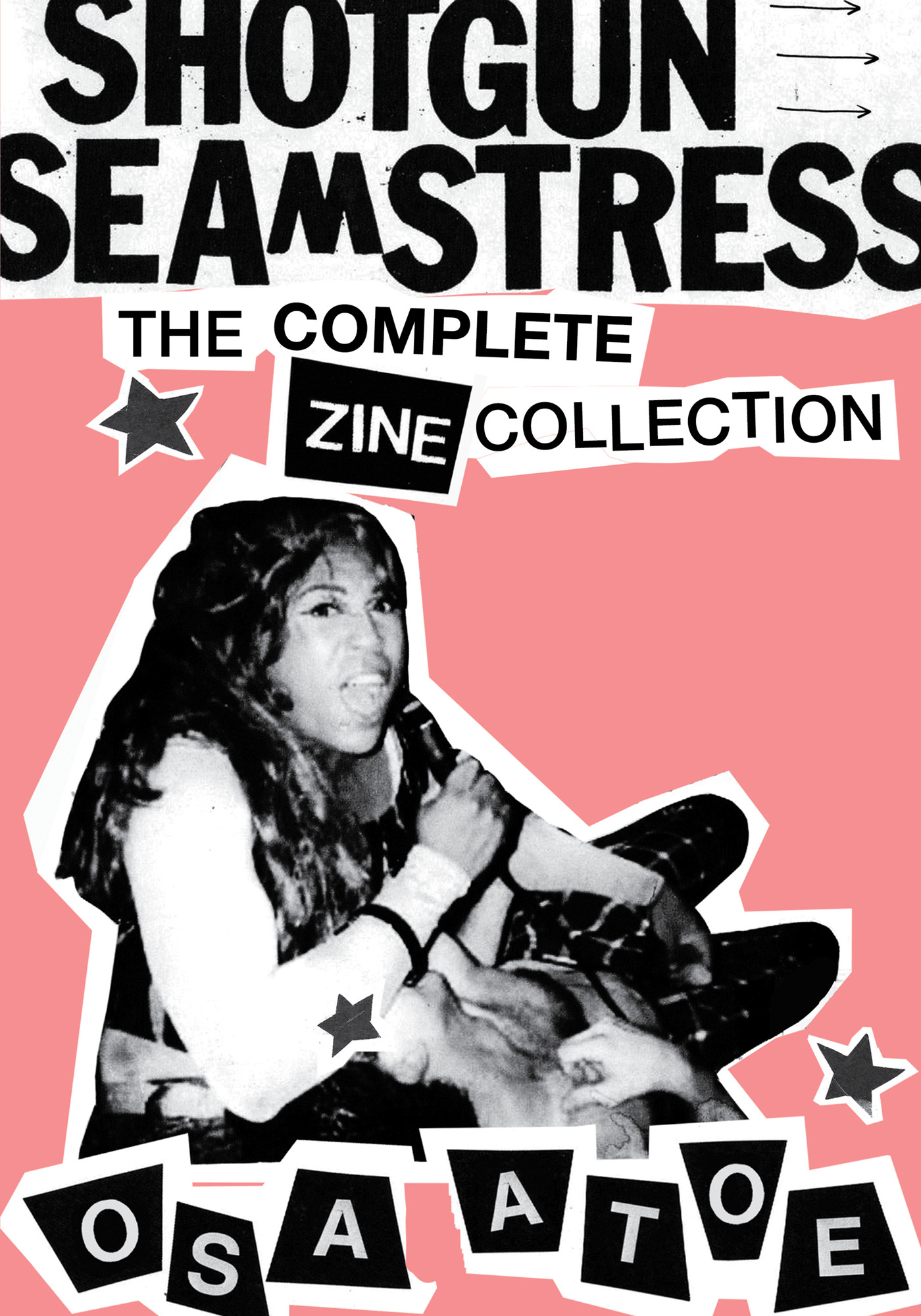This vertical rectangular poster, designed with a mix of vibrant and contrasting colors, prominently features a central image of a woman holding a microphone, appearing to sing passionately. At the top, within a neat white rectangle border, bold black letters announce, "Shotgun Seamstress." Below this, against a striking pink background, it further proclaims, "The Complete Zine Collection" in slightly smaller black letters. The woman, depicted with long black hair and wearing a vest over a shirt, occupies the bottom section of the poster. Her image is stylized with a rough white border, adding an edgy feel to the design. Notably, a pair of legs, draped casually across her lap, suggest the presence of another person. Highlighted at the very bottom, in block letters that are white on black and backed by white, is the cryptic text, "O-S-A-A-T-O-E O-S-A-A-T-O." Additionally, several black stars with white borders adorn the poster, contributing to its dynamic aesthetic.